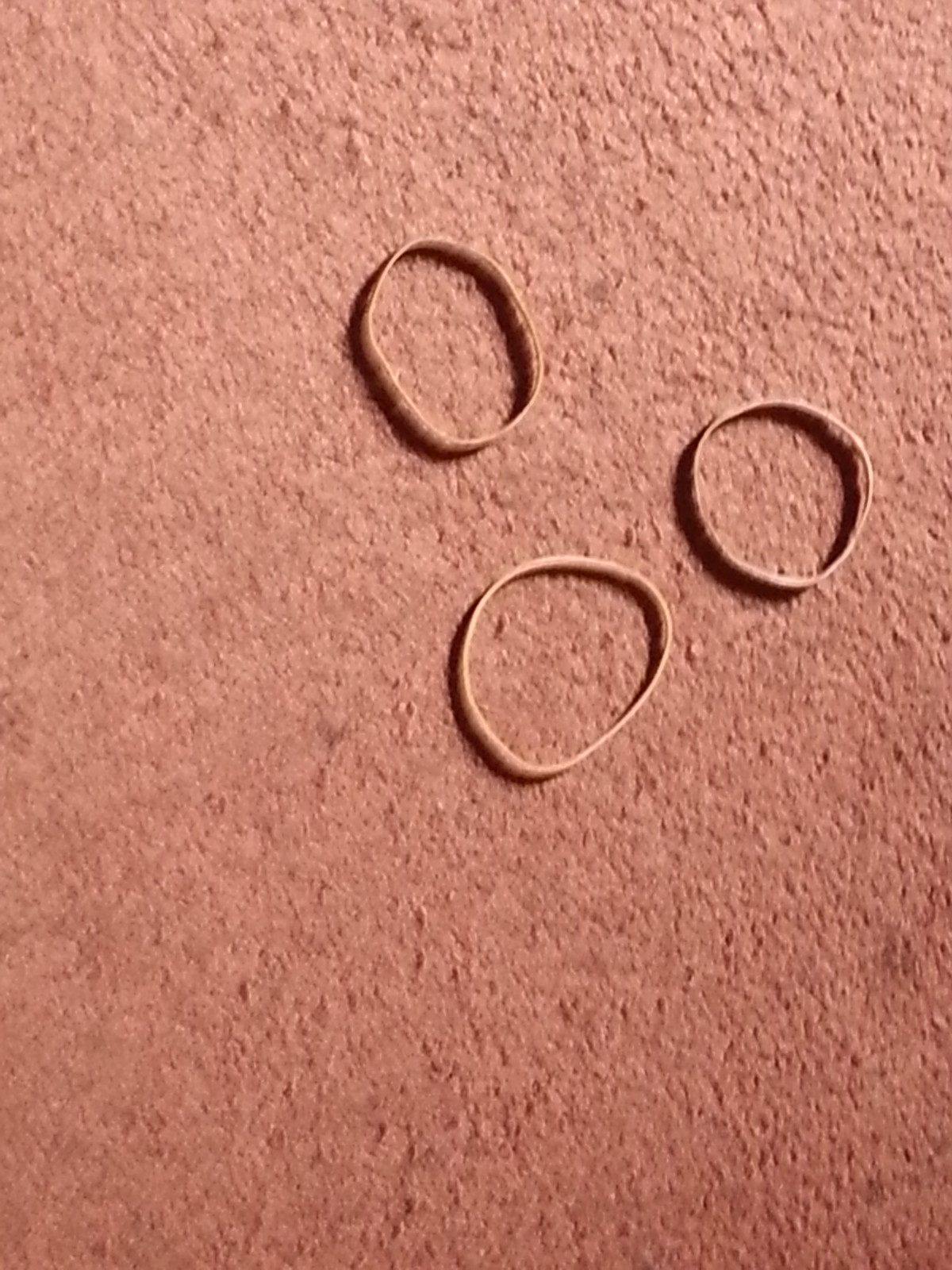This image shows three small rubber bands arranged on a red, textured background. The surface appears to have raised spots and is difficult to identify precisely due to the image's low resolution; it could be pavement or a uniquely textured carpet. The background's texture varies, being rougher on the upper right-hand side and smoother on the left, with an intermediate texture on the bottom right. The rubber bands are positioned near the center but are not touching each other. One rubber band, slightly off-center to the upper left, has an oval shape with a bump. Another rubber band is just to the right and slightly down from the center, more egg-shaped with rounded edges. The third band is closer to the right side, a bit above the center, and is almost a complete circle with a couple of bends. Shadows of the rubber bands are visible on the textured surface.